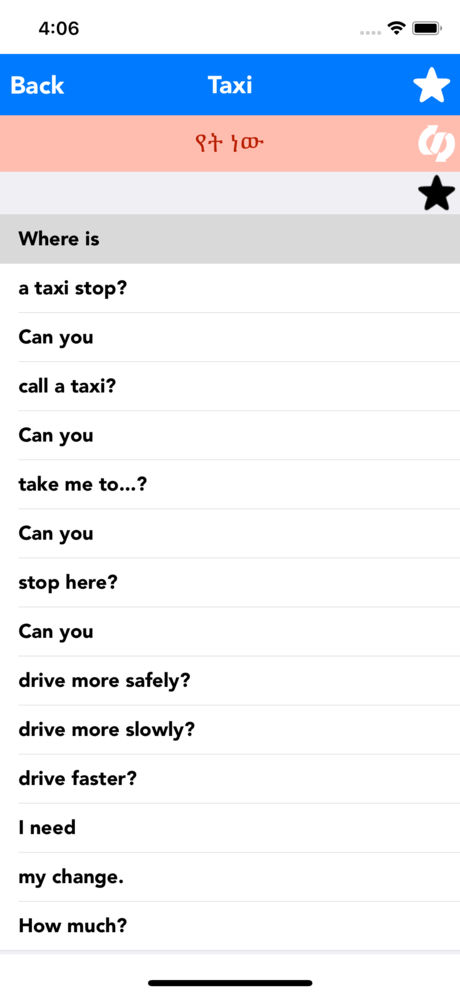This is a detailed caption for the provided image:

"Smartphone Screenshot Overview:
 
At the top of the image is a typical smartphone status bar displaying a timestamp of '4:06' on the right. Adjacent to the timestamp, there are three gray dots indicating connection strength, a strong Wi-Fi signal icon, and a fully charged battery icon.

Below the status bar, there is a blue header section with white text. The word 'Back' is aligned to the left, 'Taxi' is centered, and a star icon is positioned on the right.

The next section features a peach-colored box with red text written in an unfamiliar language, accompanied by a rightward swirly arrow icon.

Underneath, there is an empty white box with the exception of a black star located on the right edge.

Following is a gray box containing black text that indicates the current location.

Subsequently, a series of white boxes, each presenting different pre-set text options commonly used for communication in a taxi context, are listed. These options include:
- 'Taxi stop'
- 'Can you call a taxi?'
- 'Can you take me to...'
- 'Can you stop here?'
- 'Can you drive more safely?'
- 'Drive more slowly'
- 'Drive faster'
- 'I need my change'
- 'How much?'

At the bottom, a solid black line seems to represent a return to the homepage interface.

Finally, there is another box for indicating the current location, followed by the same series of questions."